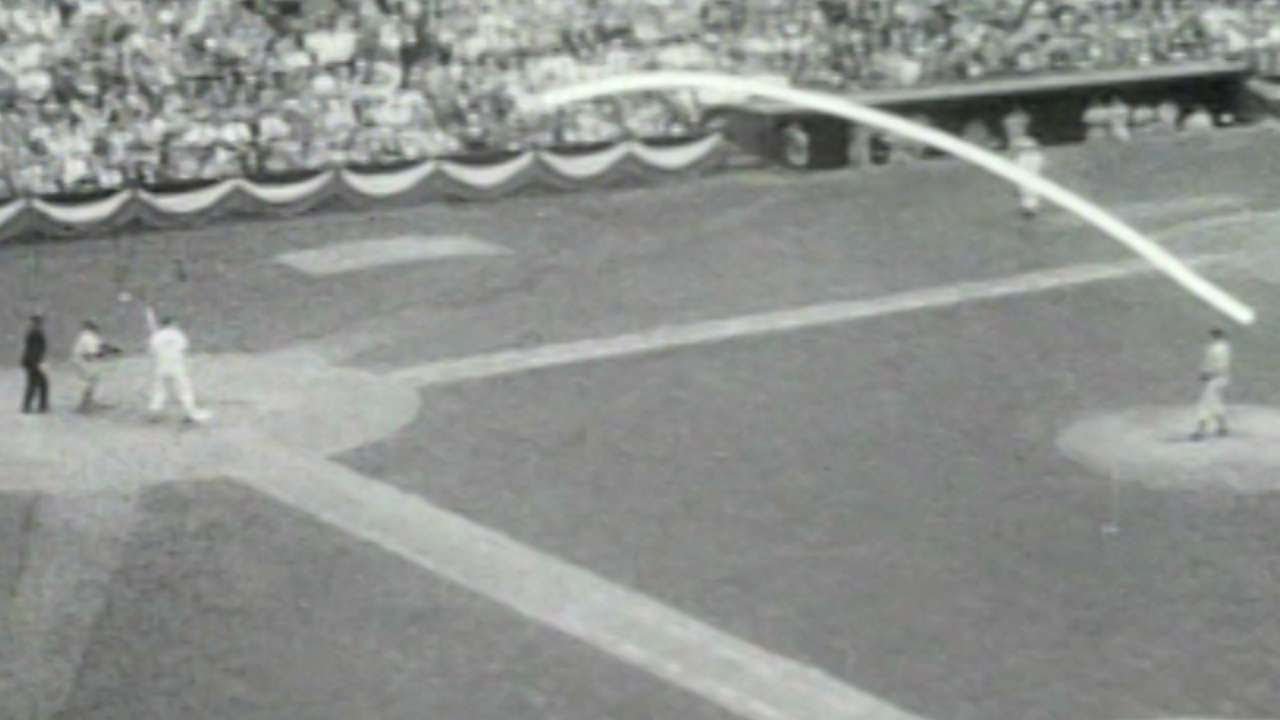The image depicts a faded, black and white photograph of a historical baseball field, likely from the mid-20th century. On the left side, the batter, catcher, and umpire are positioned near home plate, with the batter prepared to face the pitcher, who stands on the mound toward the middle right of the image, not quite in a pitching stance. A distinct, white, curved line or arrow extends from the pitcher upwards and across the field, suggesting the trajectory of a pitched or hit ball, moving towards the top right corner of the image. In the background, the stands are filled with spectators, and near the top right, the dugout is visible with additional players. The teams are distinguishable by slightly different shades of uniform, with one team in gray and the other in a lighter color. The entire scene is set on a flat field, capturing a moment in the midst of a game, steeped in the nostalgic atmosphere of an earlier era in baseball history.